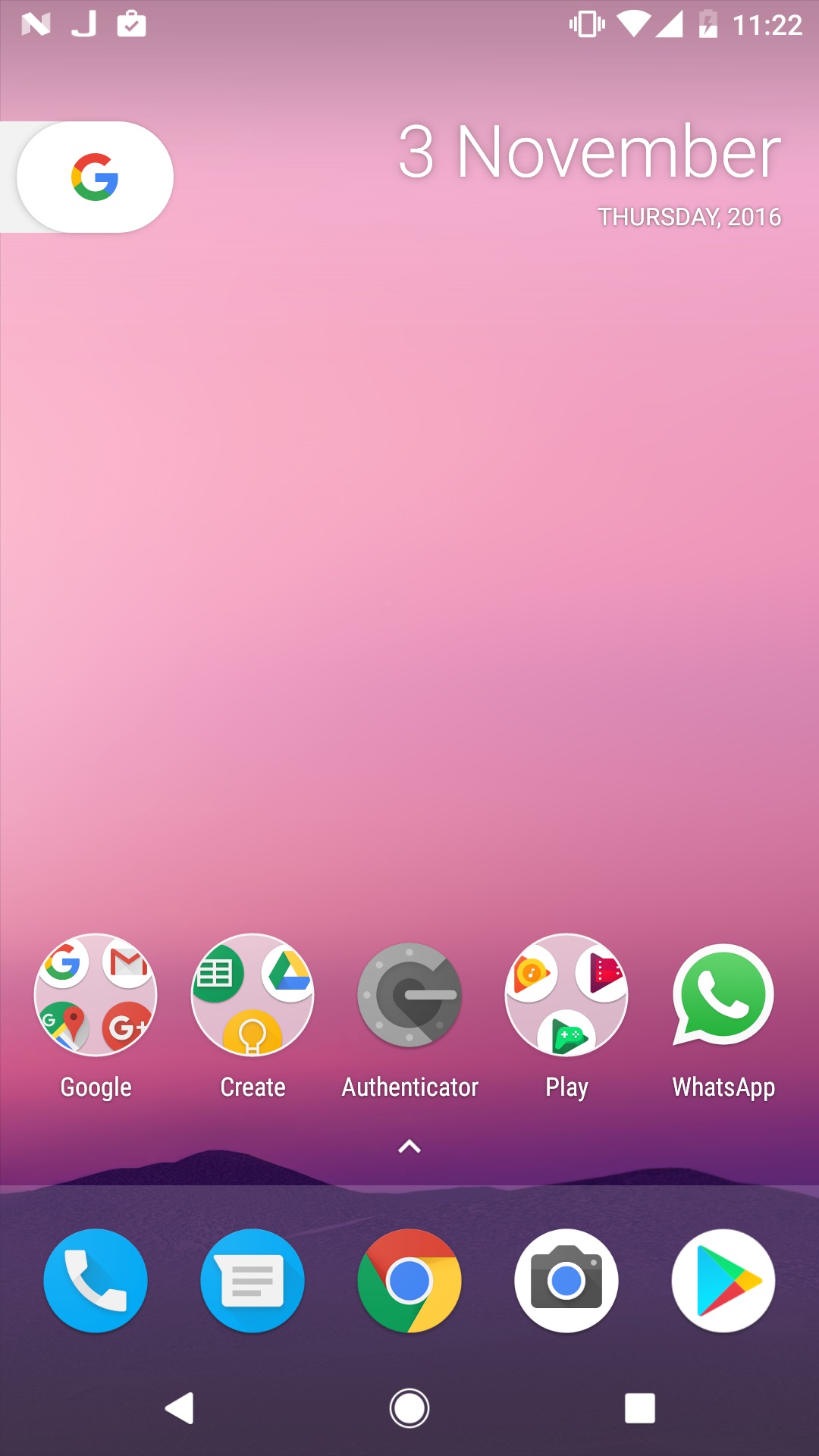This is a screenshot captured from an Android phone. In the top right corner of the screen, the time is displayed as 11:22. Adjacent to the time, the battery icon shows approximately a half-full battery, followed by Wi-Fi and vibration mode icons. The top center of the screen lists the date in large white text, "3 November," followed by the day, "THURSDAY, 2016," in uppercase letters. Near this area, towards the right, is the circular Google logo, indicative of a Google widget. 

The phone's wallpaper features a serene landscape with pinkish-purple hues and subtle hills at the bottom. Along the bottom of the screen, there are five circular application icons: Google, Create, Authenticator, Play, and WhatsApp. Below these icons, a light-gray border houses additional application icons.